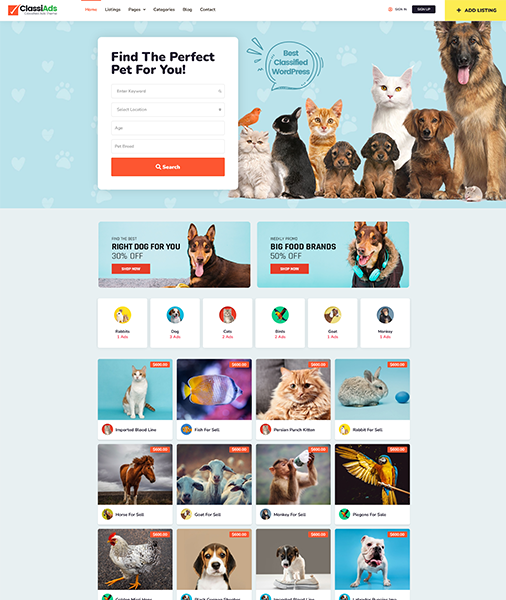The screenshot showcases a webpage from a classified ads website, designed specifically for pet listings. The website features an organized layout with various sections including "Home," "Live Page," "Listings," "Categories," "Blog," "Contact," "Sign In," "Sign Up," and "Ad Listing." The central headline reads: "Find the perfect pet for you. Best classified WordPress."

A prominent search bar invites users to enter keywords and select conditions such as age and type of pet, along with a search button. 

The upper section of the page displays images of several pets available for adoption or sale: 
- A white dog
- A black and white rabbit
- An orange cat
- Two brown and black dogs
- A white cat
- A reddish-brown dog
- A brown and black German Shepherd

Promotional banners below the pet photos advertise discounts: "Right dog for you, 30% off shop now" and "Big food brands, 50% off shop now."

Further down, round icons lead to additional information, followed by an array of other pet listings:
- A cat labeled as an "Imported Breed"
- Fish for sale
- An orange furry cat
- A gray rabbit next to a blue egg
- A brown horse
- Several white goats
- A monkey drinking from a water bottle
- A bird with its wings spread
- A white and black chicken
- A brown and white puppy
- A white and black puppy chewing on a shoe
- Another white dog

The background color of the webpage is a neutral gray, providing a clean and unobtrusive backdrop for the colorful pet images and icons.